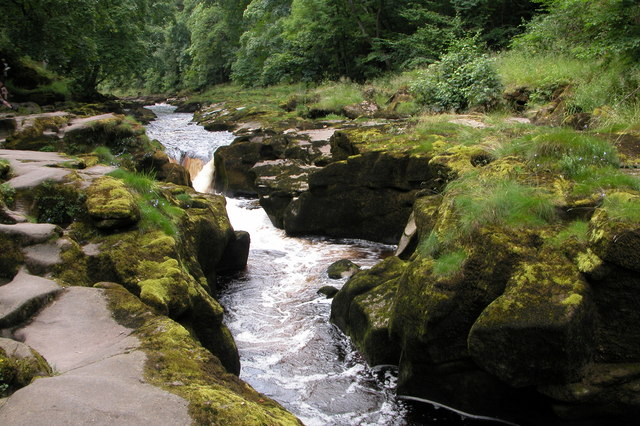An enchanting outdoor nature scene captures a serene creek meandering through a rugged, rocky terrain. The creek, with its jagged edges, flows gracefully into the dense forest, bordered by an assortment of moss-covered rocks. On the left side of the creek, a line of flat rocks forms a natural walkway, while the right side is dominated by rocks blanketed entirely in lush grass and moss. These rocks are deeper in the foreground, almost forming a barrier over the creek, but gradually become more level with the water as they recede into the background.

The landscape to the right features vibrant grassy patches that seamlessly blend into the forest, which is abundant with thick, verdant trees. The entirety of the scene is bathed in various shades of green—from the lively foliage of the trees to the rich grass and the moss that adorns many of the rocks. The creek's clear, flowing water is animated by white rapids, which sparkle under the sunlight, emphasizing the untouched splendor of this wilderness.

The forest itself, with its dense canopy and intricate play of light and shadow, appears darker and more mysterious as it stretches deeper into the background. Amidst the greenery, spots of bright and dark leaves enhance the depth and vibrancy of the scene. The overall atmosphere is one of wild, unspoiled beauty, highlighted by the interplay of sunlight and the sheer diversity of natural elements.